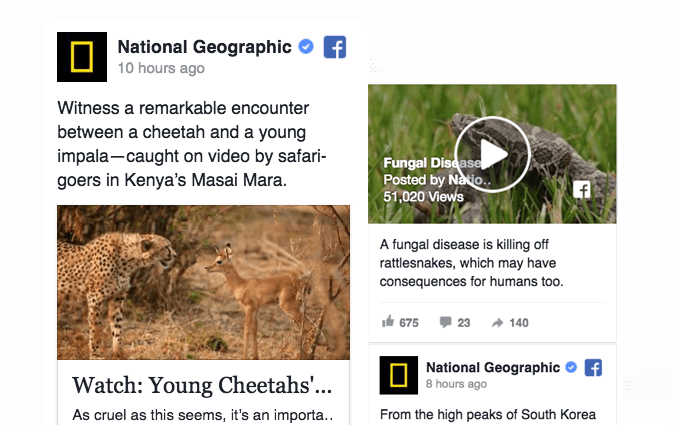Here is a revised and detailed caption for the described visual content:

---

This image appears to be a screenshot taken from either a computer or a phone. It features two distinct posts by National Geographic, both marked by a verified check mark and the Facebook symbol. National Geographic's recognizable black square logo with a yellow rectangle is prominently displayed, indicating that the posts were made 10 hours ago.

On the left side of the image, there's a post showcasing an extraordinary encounter between a cheetah and a young impala in Kenya's Masai Mara. The detailed caption reads: "Witness a remarkable encounter between a cheetah and a young impala, captured on video by safari-goers in Kenya's Masai Mara." The words "Masai Mara" are spelled out as M-A-S-A-I M-A-R-A to ensure clarity. Below this text, there is a striking photograph of a cheetah alongside what appears to be a young impala, which looks like a small deer. The caption under the image teaser says: "Watch young cheetahs... As cruel as this may seem, it plays an important role..." This is paired with a promotional video embedded within the post.

On the right side of the image, there is another post featuring a photograph of a rattlesnake. The post highlights a severe issue, stating: "A fungal disease killing off rattlesnakes may have serious consequences for humans too." This post includes statistics on the number of views and the Facebook symbol. The context and significance of this fungal disease are summarized below, drawing attention to the broader environmental and health implications.

Additionally, this post briefly references an article related to South Korea, hinting at diverse global content covered by National Geographic.

Overall, the image captures National Geographic's compelling and educational content on wildlife and environmental issues.

---